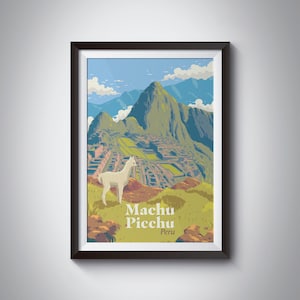The image depicts a framed poster hanging on a white wall, bathed in light. The black frame encases a white mat that borders the illustration within. At the bottom of the poster, the text reads "Machu Picchu, Peru." The illustration prominently features a white llama standing in profile on a grassy cliff in the foreground. The cliff overlooks a lush, green plateau interspersed with rocky areas and stone steps that appear to lead up towards the ancient Incan ruins of Machu Picchu in the middle ground. Though the ruins are small and lack detailed intricacy, they are set among verdant greenery, capturing the iconic essence of the site. Beyond the ruins, a vibrant green mountain range rises majestically, with further peaks fading into a lighter green and merging seamlessly with the blue sky interspersed with puffy white clouds. Overall, the illustration encapsulates the timeless beauty and grandeur of Machu Picchu, as seen from a picturesque vantage point.